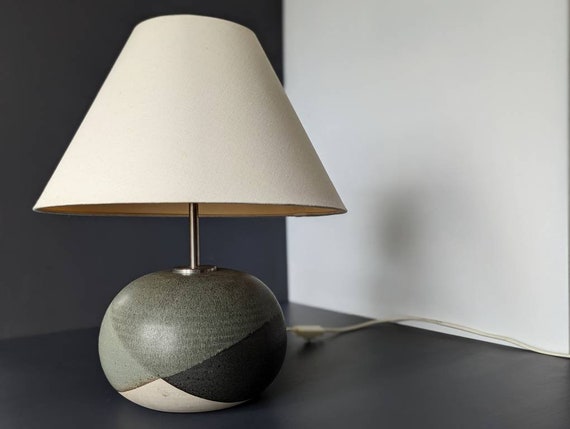This image is a color photograph in landscape orientation, showcasing a table lamp positioned on the left half of the frame. The lamp stands on an elliptical ceramic base, adorned with a geometric pattern of angled triangles in dark gray, light gray, black, and white. Rising from the center of the base is a slender metal neck supporting a triangular-shaped lampshade. The lampshade is white and gently rounded at the top, widening downwards. The lamp rests on a dark, brownish-gray wooden floor, with a dark gray wall forming the left half of the background and a white wall on the right. A white cord with a rocker switch extends from the base, trailing along the floor towards the right corner of the image. The photograph is rendered in a realistic style, capturing the intricate details and textures of the scene.